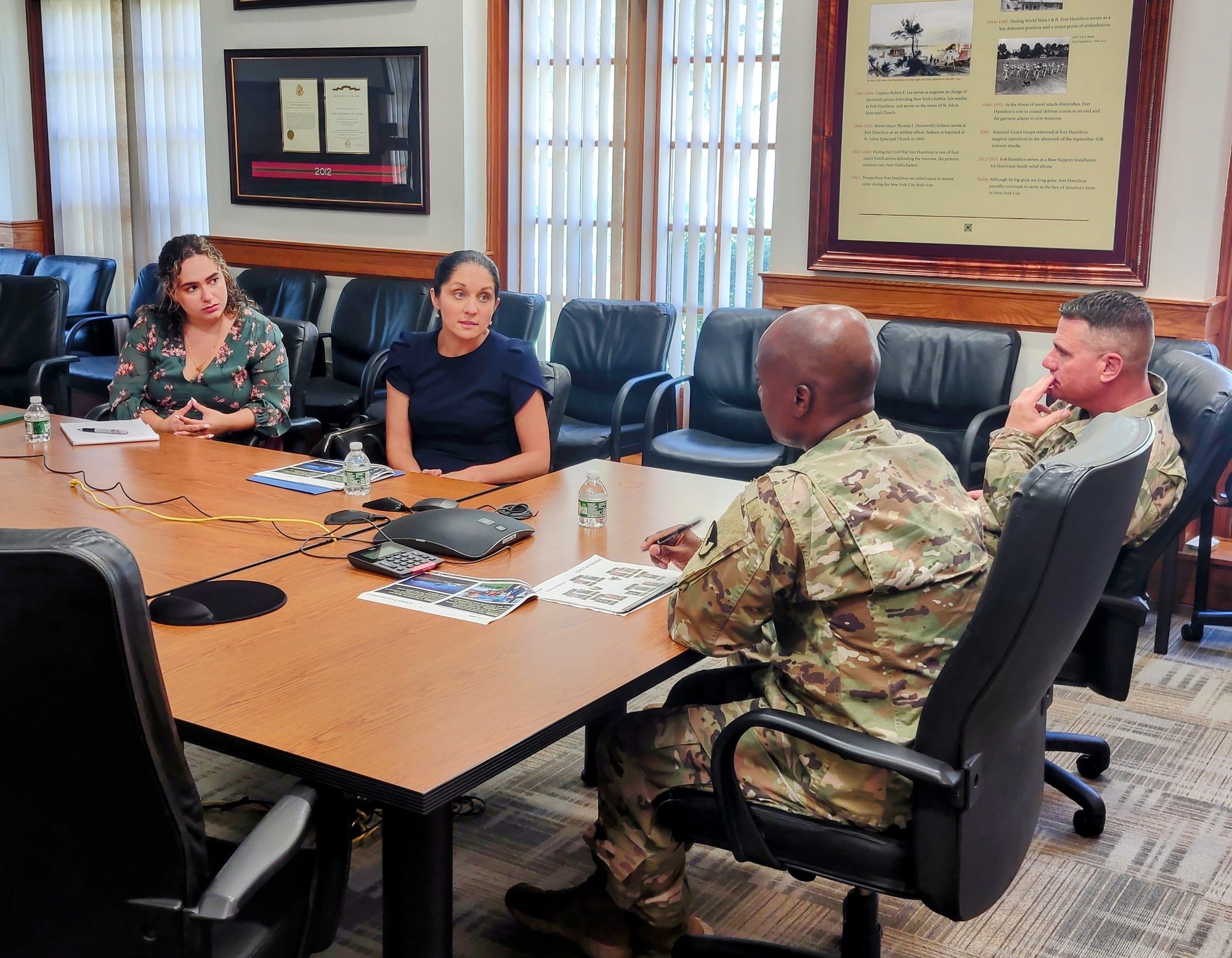In this photograph of a meeting room, we see a detailed scene of a business or military meeting in progress. The room has a long rectangular table connected to a shorter table forming a T shape, both made of brown wood, positioned in the center. Around these tables are several black leather office chairs, with additional padded blue seats along the walls. The carpeting is a tan and black striped pattern.

On the right side of the main table, two men in military camouflage uniforms are seated, one of whom is a bald black man, and the other has a marine-style haircut. In front of them are papers, a calculator, and a square black electronic device, likely for internet connectivity. Each individual has a small water bottle on the table.

On the left side near the windows, two women are seated side by side. One woman, wearing a blue blouse and having dark hair, and the other, in a flowered blouse with brown hair, are engaged in conversation with the military men. Papers are spread in front of each participant. 

The room is outfitted with several black padded chairs lined against the walls, and features two large displays that are not fully visible in detail. The walls also contain informational boards with images and explanatory paragraphs, as well as a framed picture with a black background and a red ribbon captioned "2102."

Two sets of windows with white vertical shades that are partially opened allow natural light to fill the space, enhancing visibility and adding a touch of brightness to the otherwise formal setting.